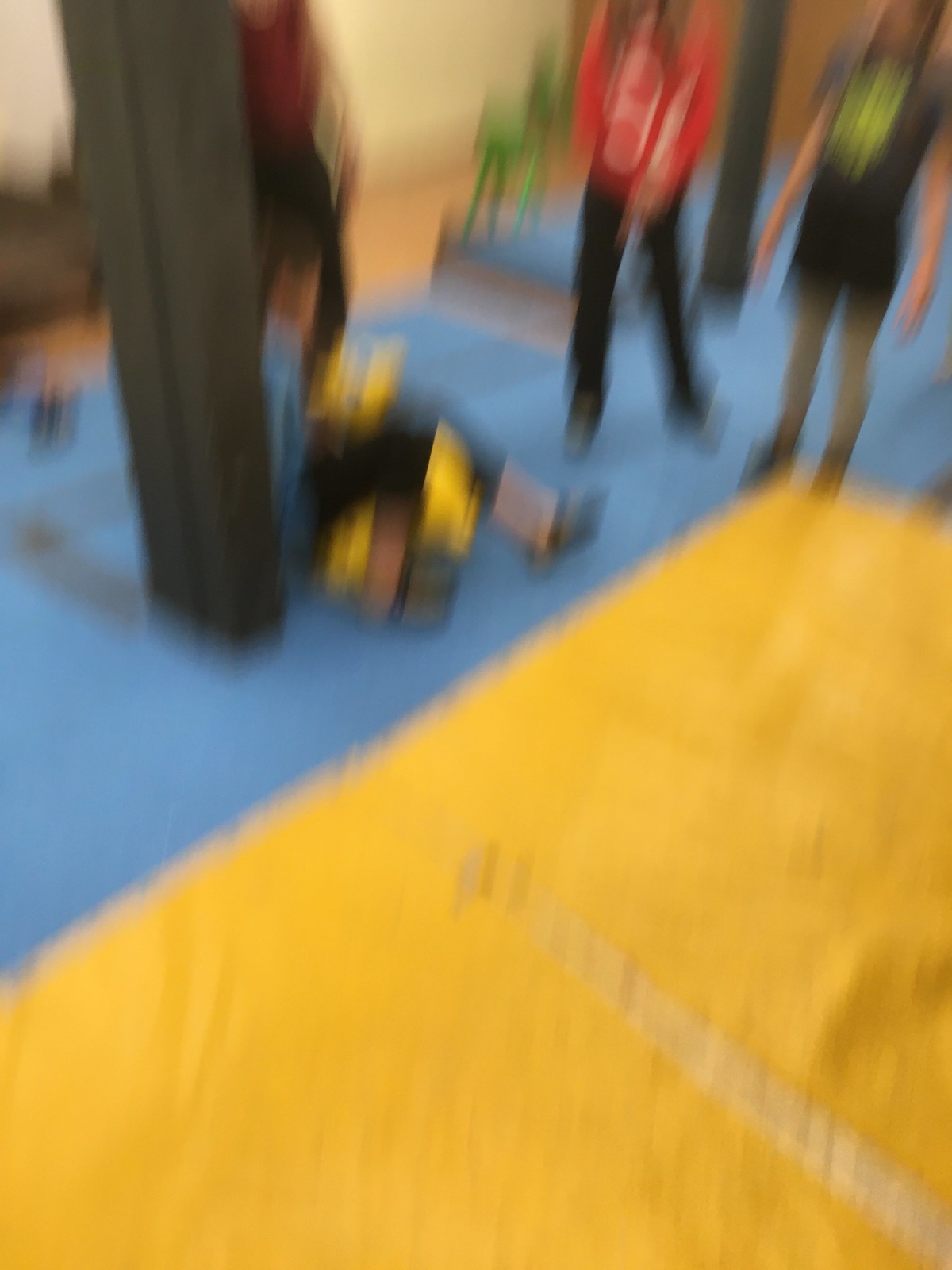This image is quite blurry, but it appears to be taken inside a brightly colored indoor facility, such as a school gymnasium or a kid's trampoline park. The flooring visible in the bottom right is a large yellow pad, which transitions into a powder blue pad as it moves up towards the center of the photo. The background shows a wall against which four girls are positioned in the blue padded area: three girls are standing while one is sitting on the floor, possibly resting or involved in an activity with the others. The standing girl on the top right has white skin and is dressed in a grayish-dark shirt with a lime green design, black shorts, gray or white leggings, and dark-colored shoes. To her left, another girl with shoulder-length hair is seen wearing a long red-sleeved shirt and black pants, while sitting directly on the blue pad, leaning against a tall black pole. This seated person wears a blue shirt and black pants, appearing to have something in their lap. Despite the blurriness, the image captures a moment of interaction among the group in the vibrantly designed space.